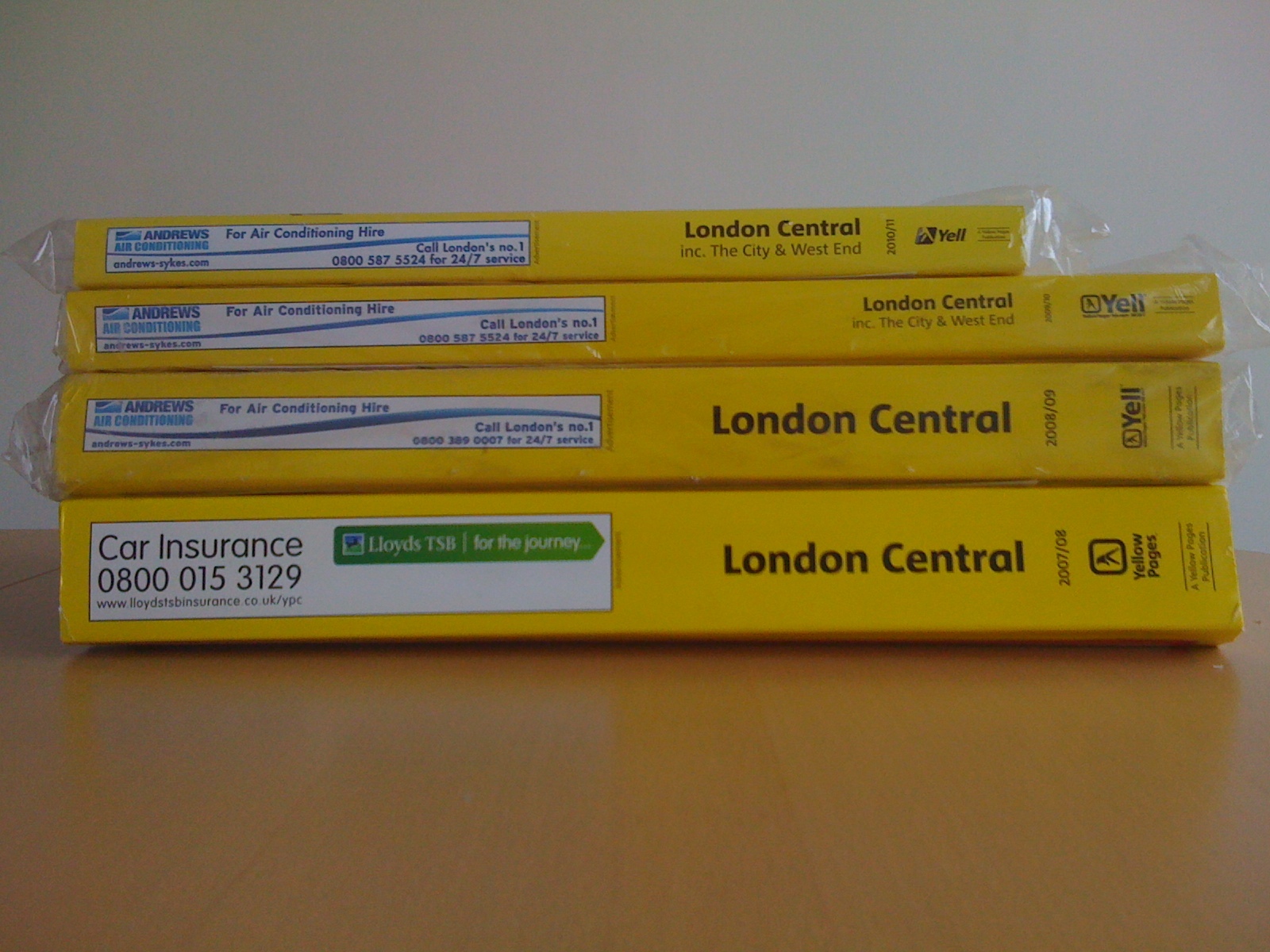The photograph captures a stack of four yellow-bound phone books, all neatly wrapped in plastic and produced by Yellow Pages for the London Central Area, including City and West End. The books are of varying thicknesses, with the largest on the bottom advertising Lloyd's Insurance for car insurance, and the three above it advertising Andrew's Air Conditioning. The top book is the thinnest and shortest. The spines feature a mix of black and white sections, with the latter containing the advertisements. Notably, the top three books have the "Yell" logo, whereas the bottom one prominently displays "Yellow Pages." The stack rests on a yellow pine table, set against a plain white wall, providing a simple backdrop to highlight the details of the phone directories.